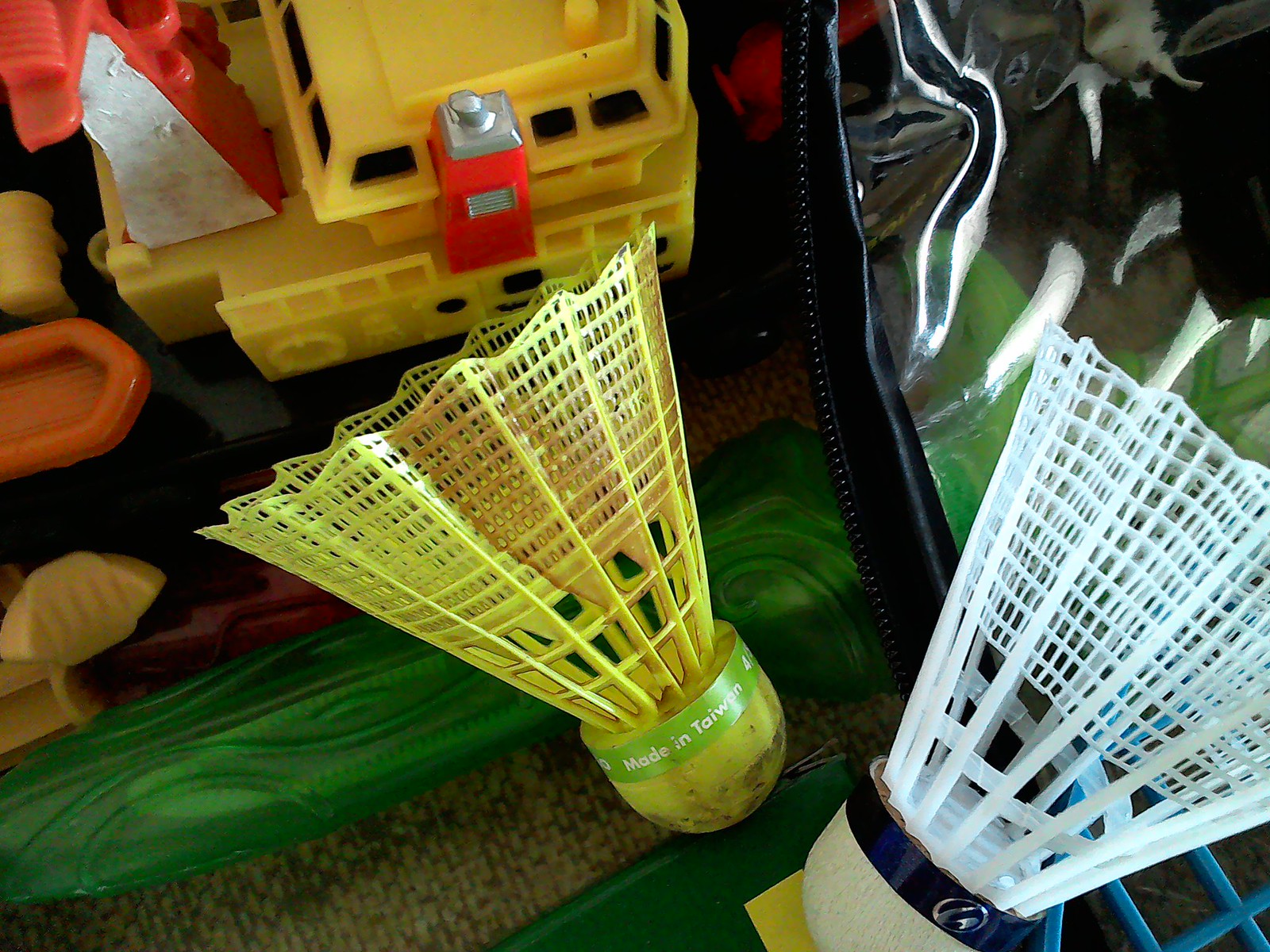In the image, we can see two badminton shuttlecocks in the foreground. The one on the left is yellow with a light green band around the base, and the one on the right is white with a dark blue ring around its base. Both shuttlecocks feature netted tails. There is some green fabric or mat underneath them, along with hints of a light brown rug. Above and to the left of the shuttlecocks is what appears to be a yellow plastic toy boat. To the right in the background, we can see part of a suitcase or container. Additionally, there is a yellow object with red, orange, and green accents visible in the background, adding a splash of color to the scene.